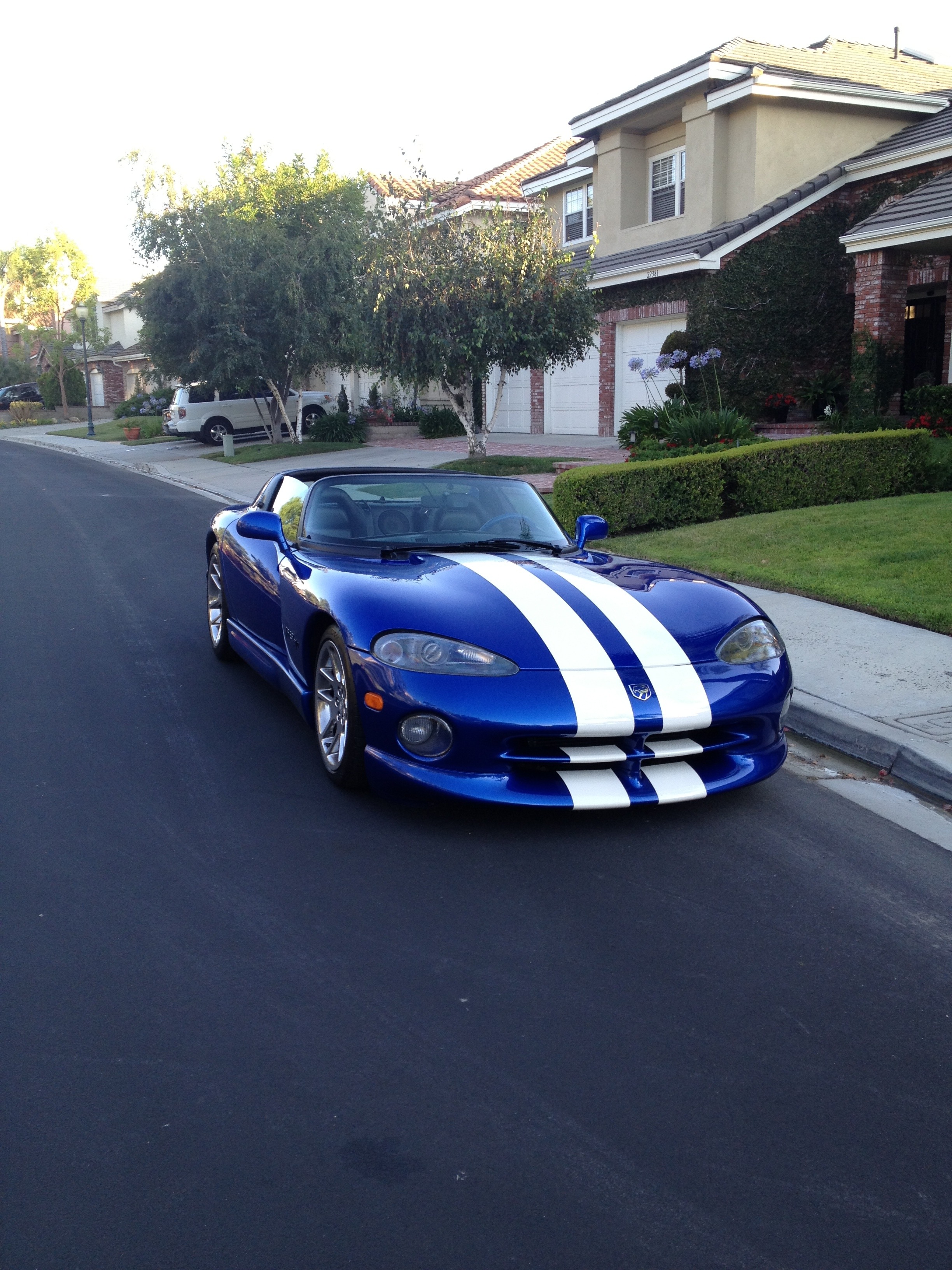This vertical rectangle photograph captures a vibrant, shiny blue Corvette with striking white racing stripes running along the hood and down the bumper. The sporty, convertible car has its top up and occupies the foreground, parked neatly at the curb on Lack Macadam Street. The right headlight is prominently visible, indicating its proximity to the curb. Behind the Corvette, a well-maintained residential neighborhood unfolds, marked by a series of attractive houses. The house immediately behind the car features a green lawn bordered by a hedge along the driveway. Adjacent to it is a larger house with a notable three-car garage and a concrete driveway, where a white SUV is parked. Taller trees dot the landscape, partially obscuring another house further down the street. The smooth, dark gray street contrasts with the lighter gray sidewalk that runs parallel. The composition of the image, with its detailed backdrop of suburban charm and the sleek, eye-catching sports car, creates a vivid portrayal of a picturesque neighborhood scene.